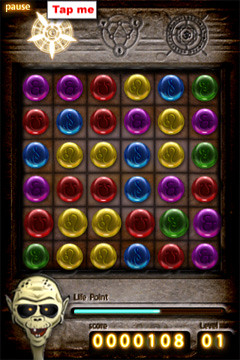This is a detailed screenshot from the Kinect 3 mobile video game. At the center of the screenshot is the main gameplay area, featuring a grid populated with a series of brightly colored circles or spheres, randomly arranged. These spheres are designed to be movable, and it appears that players need to match them in groups of three to progress in the game. 

In the bottom left-hand corner, there's a stylized image of a ghoul or Halloween creature with an oblong face, black eyes with red pupils, and a sinister smile. Adjacent to the ghoul is a light blue bar labeled "LIFE POINT," with a series of numbers displayed below it, indicating the player's life statistics.

At the top of the screenshot, red text reads "TOP ME," flanked by three symbols that extend across the playing area, likely serving as additional gameplay elements or indicators. The overall visual presentation combines vibrant colors and thematic elements to create an engaging gaming experience.